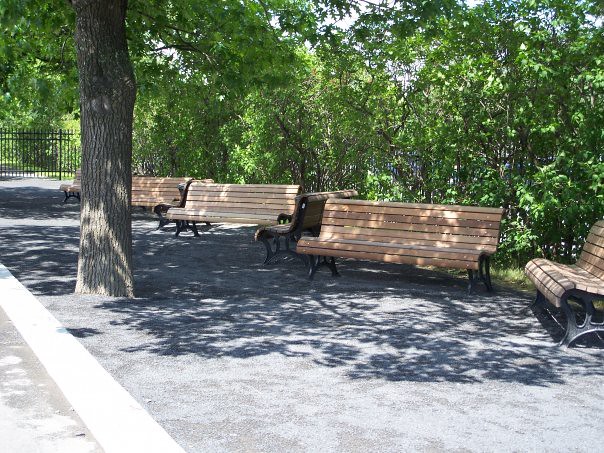An outdoor photograph captures a park area with multiple elements arranged horizontally. The scene features around seven to eight sturdy park benches, crafted from light to medium brown wood with black, ornate metal legs. These benches are positioned in a zigzag pattern along a perimeter of a gravel area, adding a dynamic visual element to their arrangement. The benches vary in orientation, facing in different directions, with some showing their armrests while others do not.

In the foreground, a large, healthy tree grows directly from the gravel, its canopy casting a network of shadows over the surroundings. The image also includes a small footpath running along the left side, and a curb outlining a cement surface where another substantial tree is planted.

The background reveals a tall, spiked, black wrought-iron fence partially obscured by smaller trees and bushes. The fence and greenery create a natural border for the park, enhancing the serene atmosphere. The photograph, though not professionally taken, offers a comprehensive glimpse into this tranquil public space dominated by greenery and well-spaced seating arrangements.